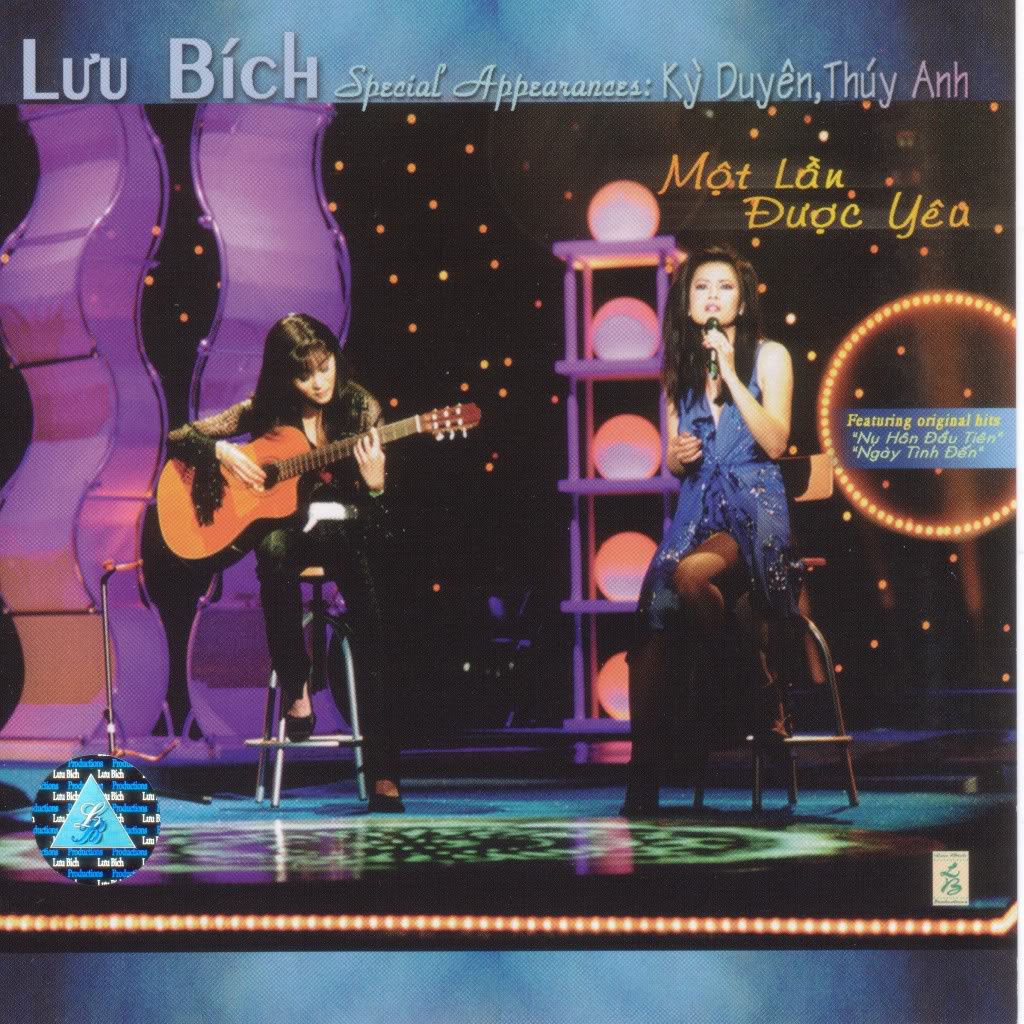This vibrant, detailed poster features two women performing on stage, capturing a dynamic and colorful scene. The performer on the left is an Asian woman with long black hair, dressed in a striking long blue gown with a high slit revealing her knee, and she is seated on a stool, singing into a microphone held close to her lips. To her right sits another woman with long black hair, wearing black pants and focused intently on playing a guitar. The stage setting includes purple pillars and white lights in the backdrop, with additional props like glowing orbs and a distinctive LED strip light along the bottom, evoking a 1990s aesthetic.

At the top of the poster, in bold text, it reads "Lu Bich," followed by "Special Appearances: Ky Duyen, Thuy Anh" and other names. A round highlighted circle includes the text "Featuring Original Hits," and there are additional lines in a foreign language. The entire scene is framed with a blue border, and the color palette includes various shades of blue, black, purple, pink, green, yellow, and tan, highlighting the overall lively and engaging atmosphere.